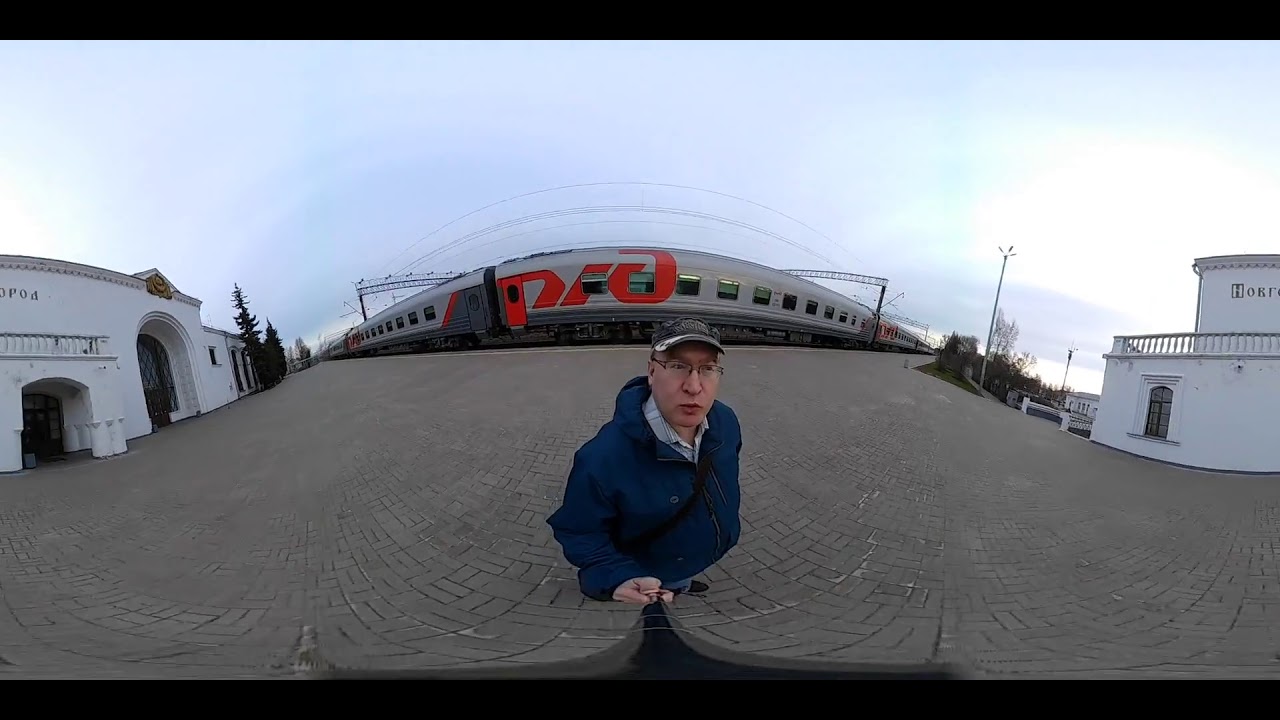In this 360-degree panoramic shot, we see a man in his 40s taking a selfie with a heavily distorted selfie stick, reflecting the unique perspective of the photograph. He is wearing black-framed glasses, a gray baseball cap, a blue coat, and blue jeans, with a gray or white undershirt. Behind him stretches a long, gray passenger train marked with red letters "P.I." or "P.I.D.," adding to the depth of the scene. The railway station platform he stands on is made of gray bricks and features buildings on both sides. The white buildings have a somewhat European or South American architectural vibe and contain distinct black lettering: "O.E.T." and "P.O.D." The building on the left has a large archway, while the one on the right features a white balcony and potentially a widow's walk. The curved distortion of the 360-degree lens makes the landscape bend downward at the edges, adding a surreal aspect to the scene. The sky above is a whitish blue, creating a crisp, daylight backdrop to the outdoor setting.